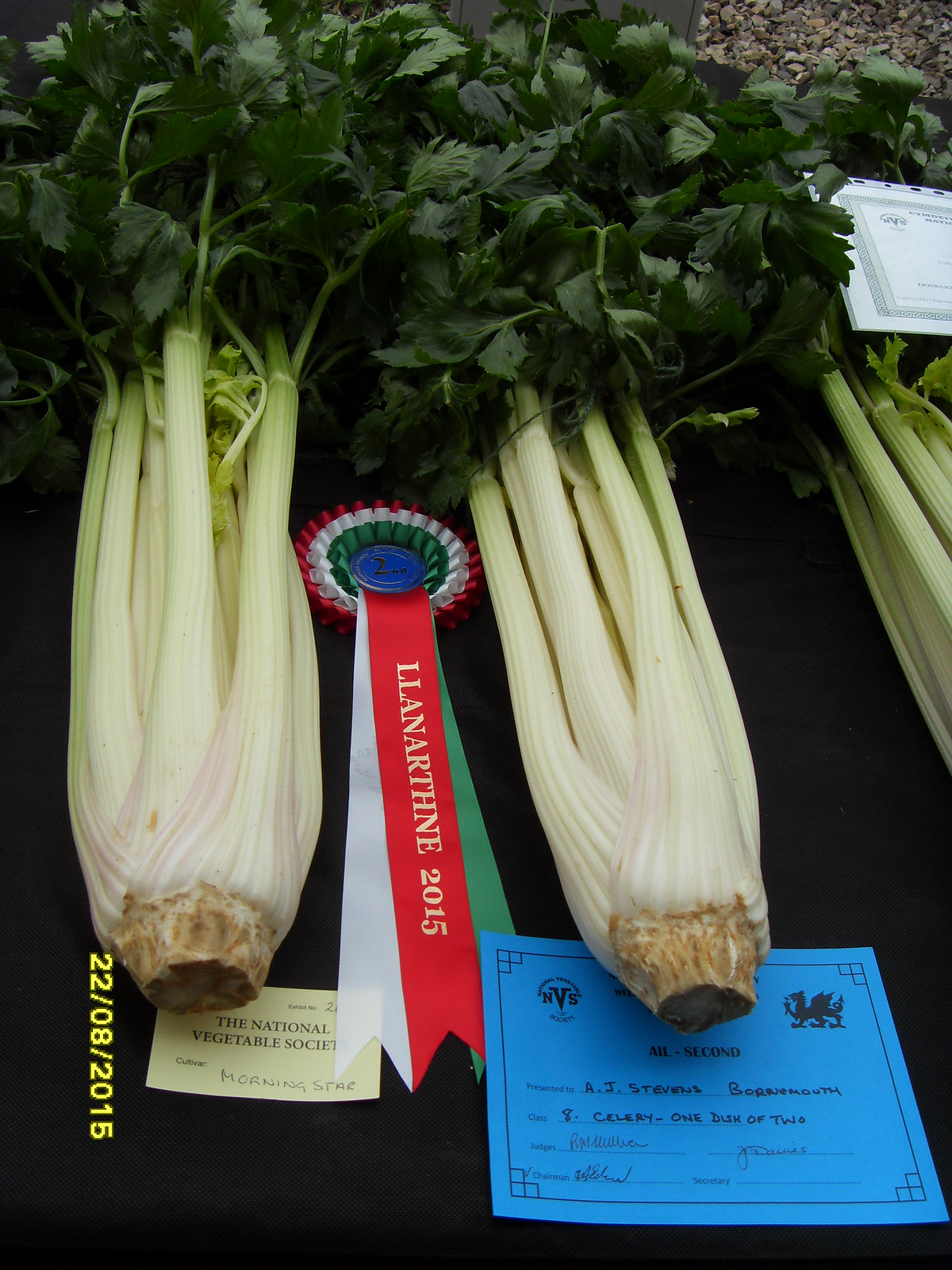This full-color photograph, timestamped August 22, 2015, captures a detailed scene at a county fair. Displayed on a table draped with a dark cloth, likely black or dark blue, are three full stalks of celery. The leftmost celery stalk is accompanied by a little white card bearing the text "The National Vegetable Society" and a ribbon indicating it won second place at the Yelanthi 2015 competition. This ribbon is primarily red, green, and white, adorned with a blue center. Behind the middle celery stalk, there is a blue card printed with text that is difficult to read. The final stalk of celery, positioned on the far right, lacks any accompanying card or ribbon. The table is set against the backdrop of the fair, though the image focuses tightly on the vegetable display.